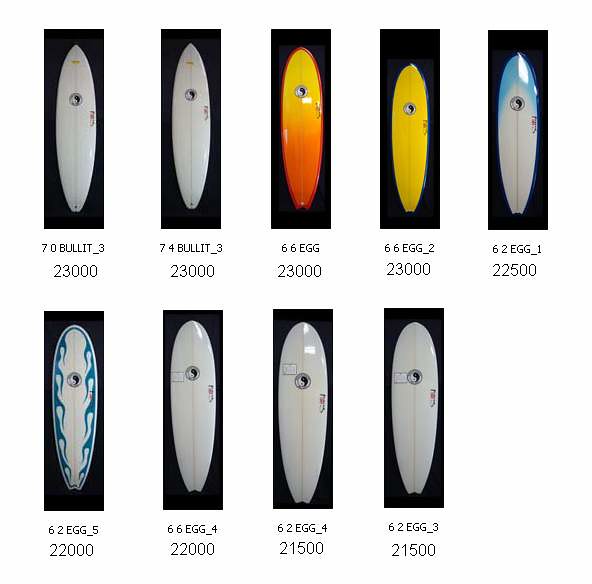The image displays a collection of nine surfboards, arranged on a black background in two rows—five on the top and four on the bottom. Each surfboard is showcased within its own rectangular frame and has a label beneath it. The labels feature what appear to be model names and prices, with most of the top row displaying "23,000" except for the rightmost one, which shows "22,500." In the bottom row, two boards are labeled "22,000," while the other two are "21,500." 

The surfboards vary in design and color. Five of them are predominantly white. Some feature distinct color transitions or patterns: one has an orange base fading into yellow, another is entirely yellow, one exhibits a white center with a blue gradient at the top, and another has a white center accented by blue waves around it. Notably, each surfboard includes a yin-yang symbol near the top.